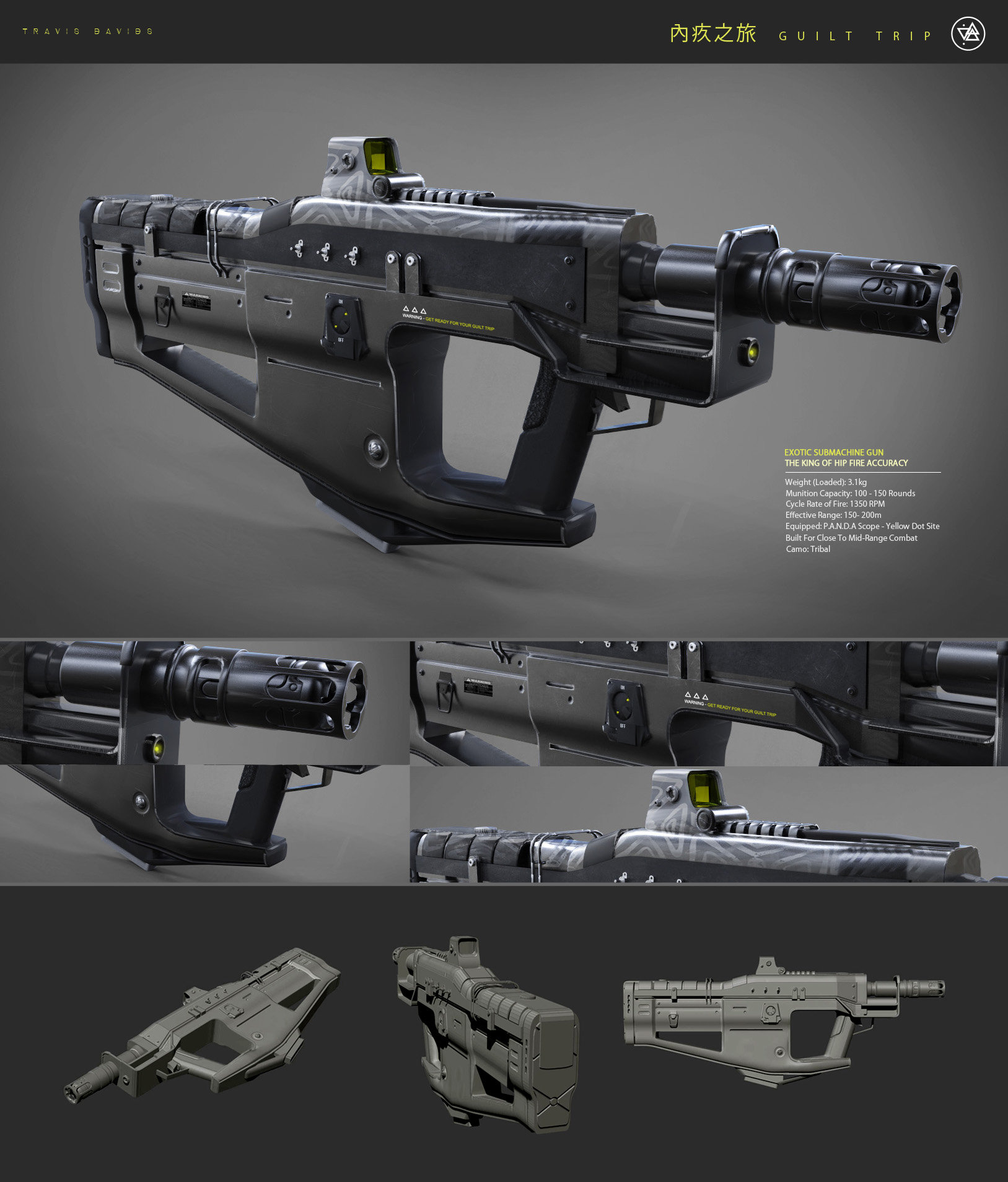This computer-generated graphic presents a highly detailed, realistic depiction of an assault-style tactical rifle. The main section at the top showcases the full length of the rifle prominently within a large rectangular frame, emphasizing its sleek, modern design. The firearm, predominantly matte black with subtle gray accents, is equipped with a green or red dot sight, enhancing its tactical appearance. Below this central image, several smaller rectangular graphics highlight specific components of the firearm: the barrel, the handle, and the optics. Additionally, the bottom section of the graphic offers various angled views of the rifle, providing a comprehensive visual understanding. The entire composition is set against a dark gray to almost black background, which enhances the contrast and detail of the firearm.